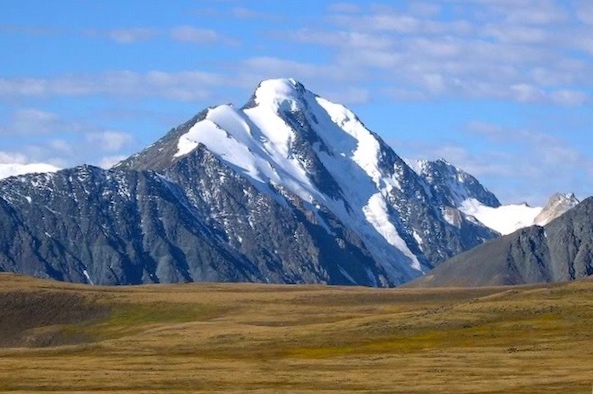The photograph showcases a majestic and imposing triangular-shaped mountain dominating the center of the image, its gray peaks notably free of vegetation and capped with snow. Patches of snow adorn the central, left-most, and right-side slopes, while an adjacent brownish-gray mountain stands to the far right. Surrounding the mountains is a flat, expansive, brownish field devoid of significant vegetation, though it may contain slight grassy patches. This field features sections of darker brown and a distinct downward indentation on the left, with a minor hilltop rising amid the sunken terrain. The sky above is blue, decorated with scattered, grayish clouds that lend a slight darkness to the scene. In the distance, a mountain range extends across the backdrop, contributing to this serene outdoor landscape devoid of any human or animal presence.